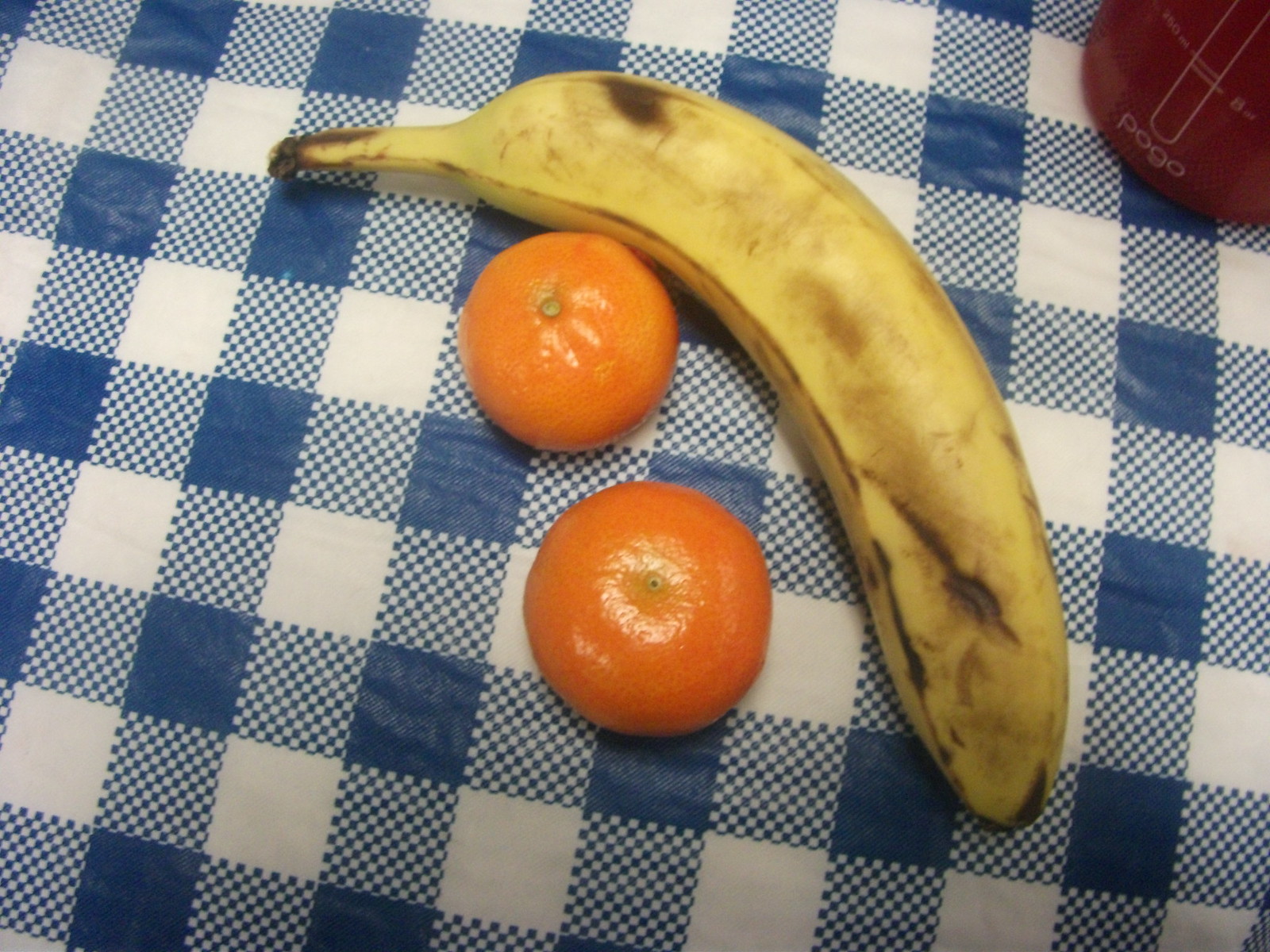This photograph captures a still life composition featuring three pieces of fruit: a heavily bruised yellow banana and two deep orange-colored oranges, all resting on a white and blue checkered tablecloth. The banana exhibits several imperfections, including pockmarks, dimpling, a brown gash towards the bottom, and bruising along the top portion. The oranges display a slight discoloration with lighter orange patches and small grayish circles at their centers. In the background, at the corner of the image, a red object with white text reading "P-O-G-O" is partially visible, adding a contrasting element to the otherwise simple arrangement. The light reflection on the fruit adds a subtle, natural shine to the scene.